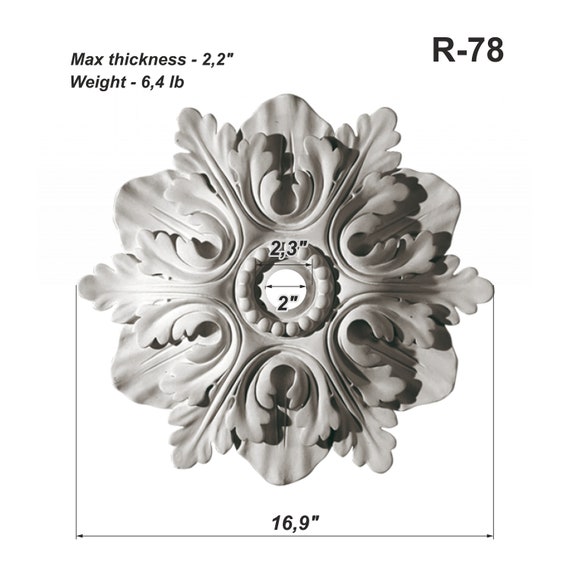The image displays a detailed rendering of a decorative ceiling medallion, likely made from plaster, ceramic, or marble. It features a symmetrical design with twelve points radiating outward, combining elements of petals and leaves. The medallion is all white, with an intricate floral motif comprising six leaf-shaped lobes and six rounded star-like points. At the center of the medallion is a circular opening, designed to accommodate a light fixture or a fastener, measuring 2 inches in diameter and labeled by arrows. Surrounding this central hole is a smaller rim measured at 2.3 inches. The overall diameter of the medallion is noted at 16.9 inches, indicated by horizontal arrows at the bottom of the image. Accompanying text on the stark white background provides additional specifications: in the top left corner, it reads "max thickness - 2.2 inches" and "weight - 6.4 pounds"; in the top right corner, it states "R-78." The text is in black font, providing a clear and precise description of the dimensions and weight of the item, which likely serves as a decorative embellishment for a ceiling light.